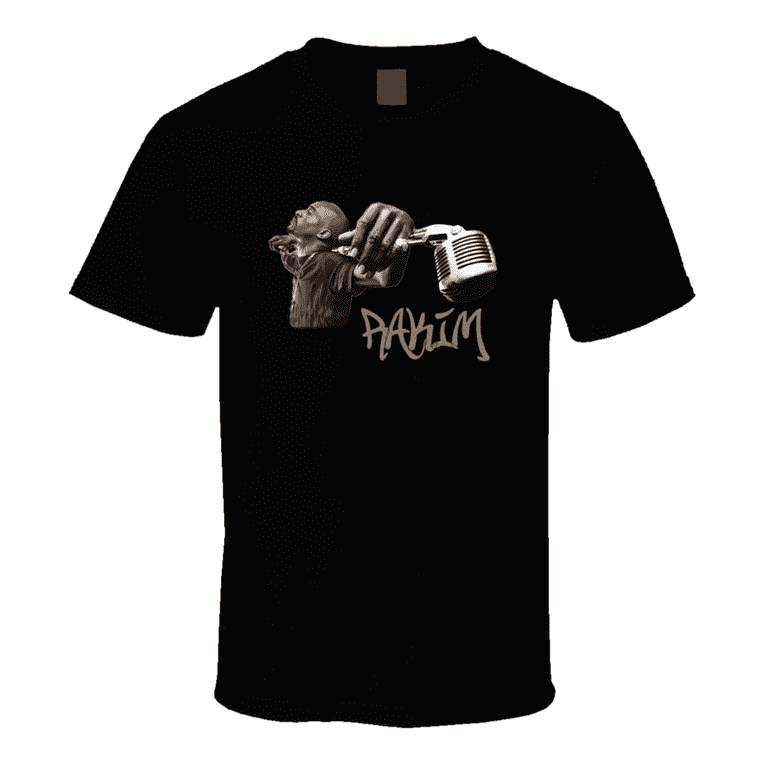The image features a black graphic t-shirt with a short-sleeve, crew neck design, set against a plain white background with no visible borders. A rectangular label can be seen on the back of the collar. The main graphic on the front of the t-shirt depicts a bald African-American man with a goatee and mustache. Positioned to the left side of the shirt, the man faces and points left, resting his arms over an old-style metallic microphone stand that stretches across the back of his neck and shoulders. His hand, with three to four fingers clearly visible, drapes over the shaft of the microphone. Below this detailed illustration, in a beige street-art style font, is the name "Rakim." The image captures the essence of a vintage recording artist, blending nostalgia with modern streetwear aesthetics.